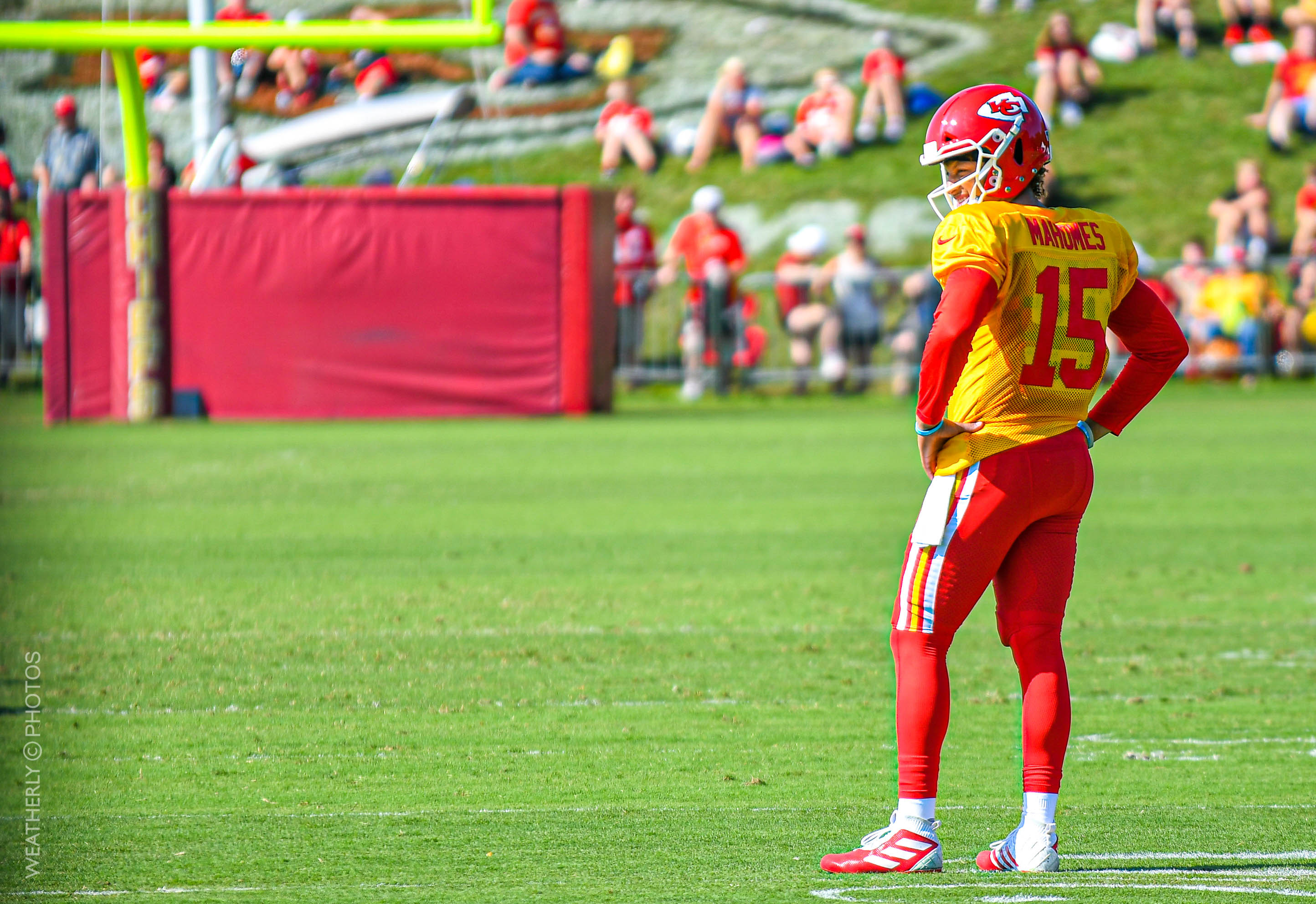This action shot captures the Kansas City Chiefs quarterback, Patrick Mahomes, standing alone on a football field. He is dressed in a vibrant yellow jersey with red type, displaying his number 15 and the name "Mahomes" across the back. Underneath, he wears a long-sleeved red shirt, which complements his red spandex pants that feature yellow and white stripes down the sides. A white towel hangs from his left side, and blue wristbands adorn his wrists. His cleats are red and white, matching his socks, and his red helmet is emblazoned with the Kansas City Chiefs arrowhead logo, featuring white and red lettering. Mahomes stands on green grass, hands on his hips, looking to the left of the image. In the background, the yellow goalpost stands prominently in front of a red wall, with spectators dressed in red and white. The scene includes people sitting and standing on an elevated grassy area, separated from the field by a barricade. The atmosphere is accented by the presence of a logo on the field and a watermark in the bottom left corner that reads "Weatherly Photos" in white text circled.